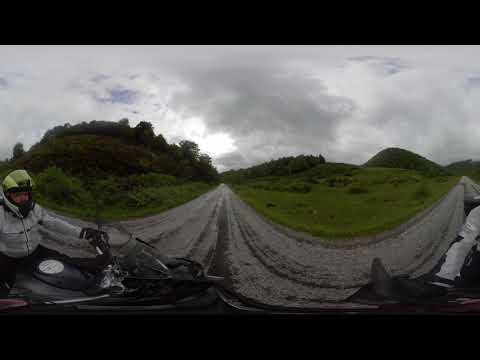In this detailed photograph taken outdoors during daytime, a motorcyclist, clad in a green helmet and a white jacket, rides a black motorcycle on a gray, winding dirt road. The road seems to curve unusually, possibly due to a panoramic camera effect. The scene surrounds the motorcyclist with green grass and trees, set against a hilly background. The sky overhead is predominantly cloudy with hints of light peeking through occasional breaks, suggesting an imminent rain. The image, appearing slightly distorted as if viewed through a car windshield, captures the motorcyclist centrally, juxtaposed against the sprawling natural scenery, conveying a sense of movement and rural tranquility.